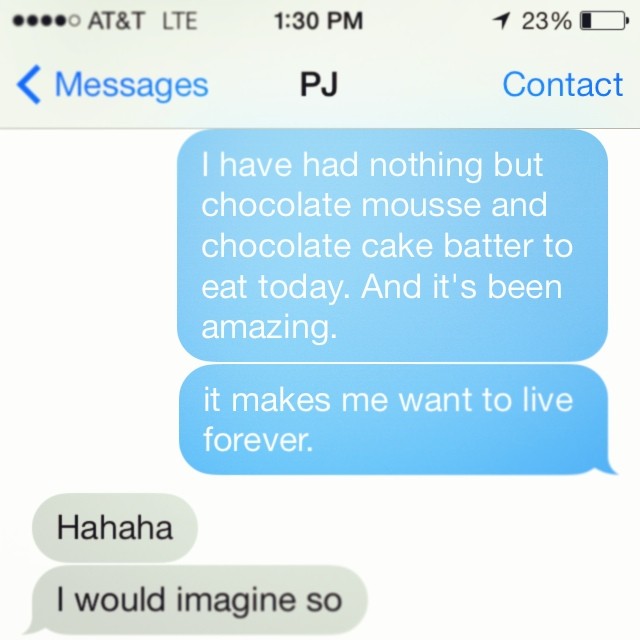The image depicts a screenshot of a text message exchange on a smartphone with AT&T service at 1:30 PM and 23% battery life remaining. At the top, "Messages" and "Contact" are visible, along with a back arrow and the initials "PJ" indicating the contact. The conversation shows two messages in blue text bubbles—"I have had nothing but chocolate mousse and chocolate cake batter to eat today, and it's been amazing. It makes me want to live forever"—followed by a response in gray text bubbles saying "Ha, ha, ha, I would imagine so." The overall background is white, and the text lacks proper punctuation and capitalization, common in casual texting.